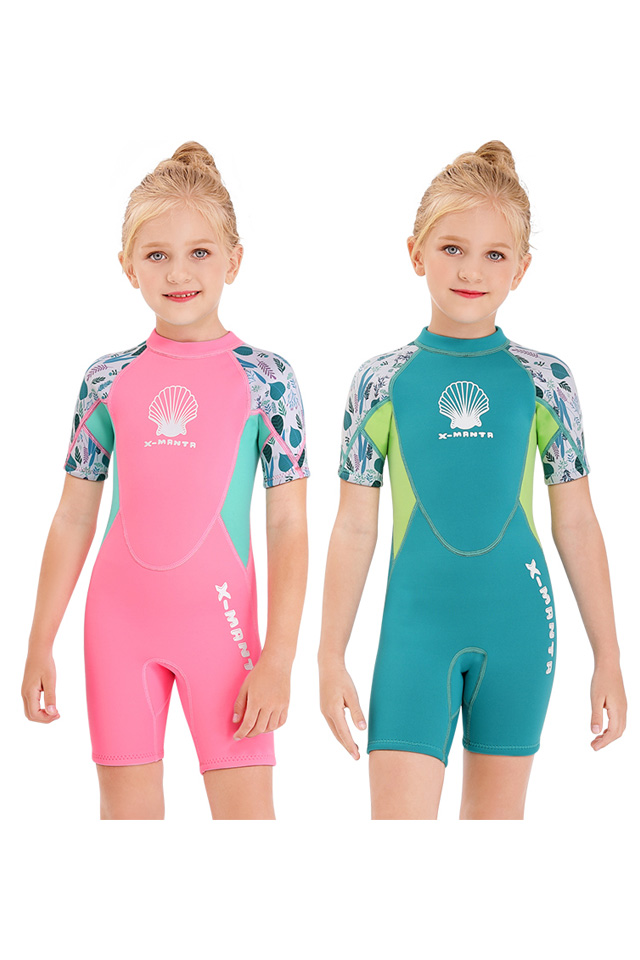The image features two young Caucasian girls, likely twins or possibly the same girl pictured twice, modeling wetsuits. The background is a stark white, emphasizing the vibrant colors and details of their outfits. Both girls have blonde hair styled in buns and noticeably red lips, with blue eyes highlighting their features. The wetsuits are short-sleeved and cut off just above the knees, suggesting they are designed for activities like swimming, scuba diving, or surfing. 

The girl on the left wears a predominantly pink wetsuit with teal highlights and a floral design on the white sleeves. She smiles softly at the camera. The chest of her wetsuit bears a logo of a white seashell and the brand name "X-Manta."

The girl on the right is dressed in an aqua blue wetsuit with lime green highlights and a similar floral design on the sleeves. Unlike the girl on the left, she has a more neutral expression. Her wetsuit also features the white seashell logo and the brand name "X-Manta."

Overall, the image appears to be an advertisement for X-Manta wetsuits, showcasing their vibrant, youth-focused aquatic apparel in a clean, minimalistic photo setting.